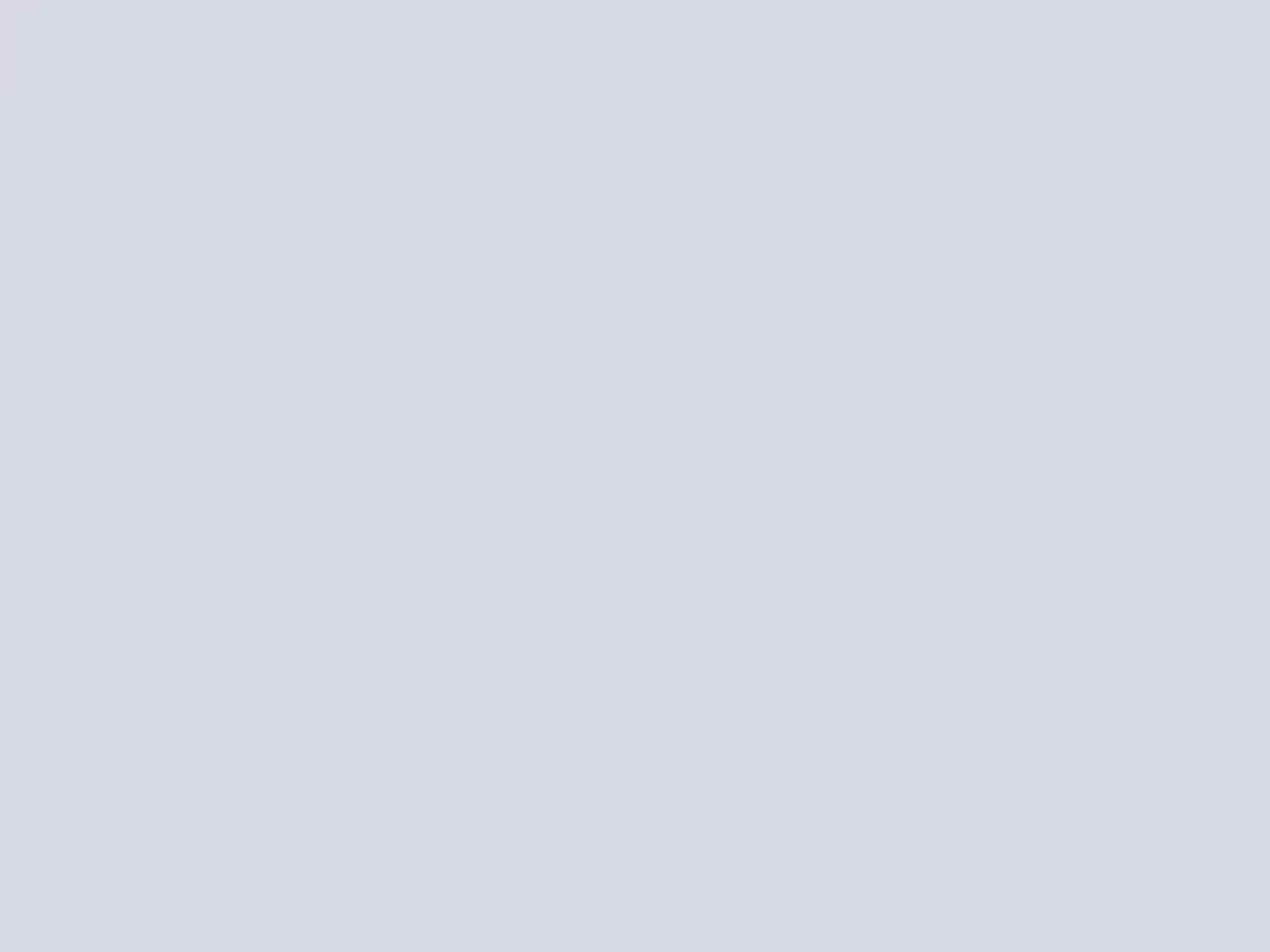This image portrays a square canvas with sharp, defined edges and corners. The primary color is a light, primer gray, featuring subtle variations with darker areas scattered throughout the center and around the edges. Several white or lighter spots are noticeable across the entire surface, contributing to a nuanced texture. The finish of the canvas is uniformly matte, lacking any glossiness. The overall effect suggests that this may be a heavily cropped close-up photograph of a painted surface or canvas, emphasizing the intricate play of light and texture on its surface.